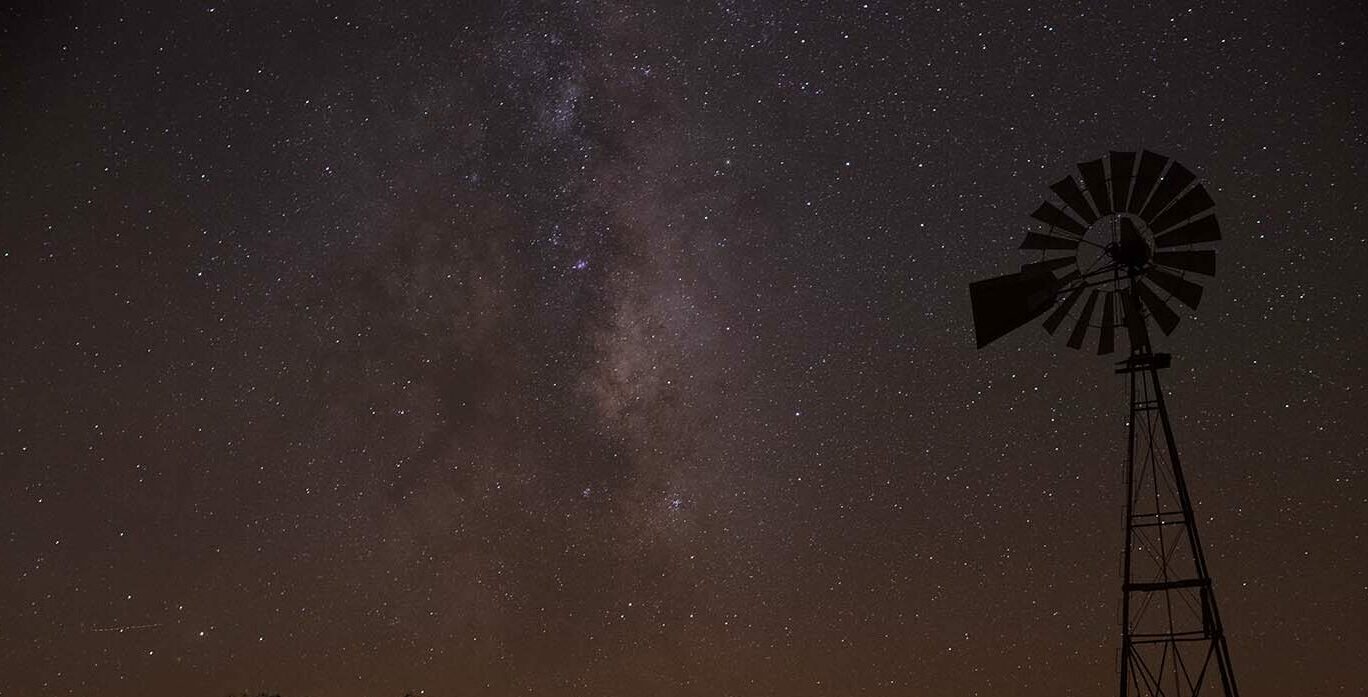The image showcases a striking night sky, filled with a myriad of stars, among which the Milky Way is distinctly visible. The background is predominantly dark, with shades of black and deep blue punctuated by clusters of stars, and a faint, lighter area running through the center, characteristic of the galaxy. On the far right side of the image stands a tall, old-school windmill atop a metal tower, which starts from the very bottom and reaches up around three-fourths of the way to the top. The windmill's silhouette is stark against the sky, with its triangular blades clearly defined. There's an intriguing detail within the windmill structure—an indistinct shape that resembles a figure holding something, adding a mysterious element. The overall scene is bathed in an ethereal, almost surreal mix of black, white, purple, and tan hues, creating a sense of serene isolation and timelessness.